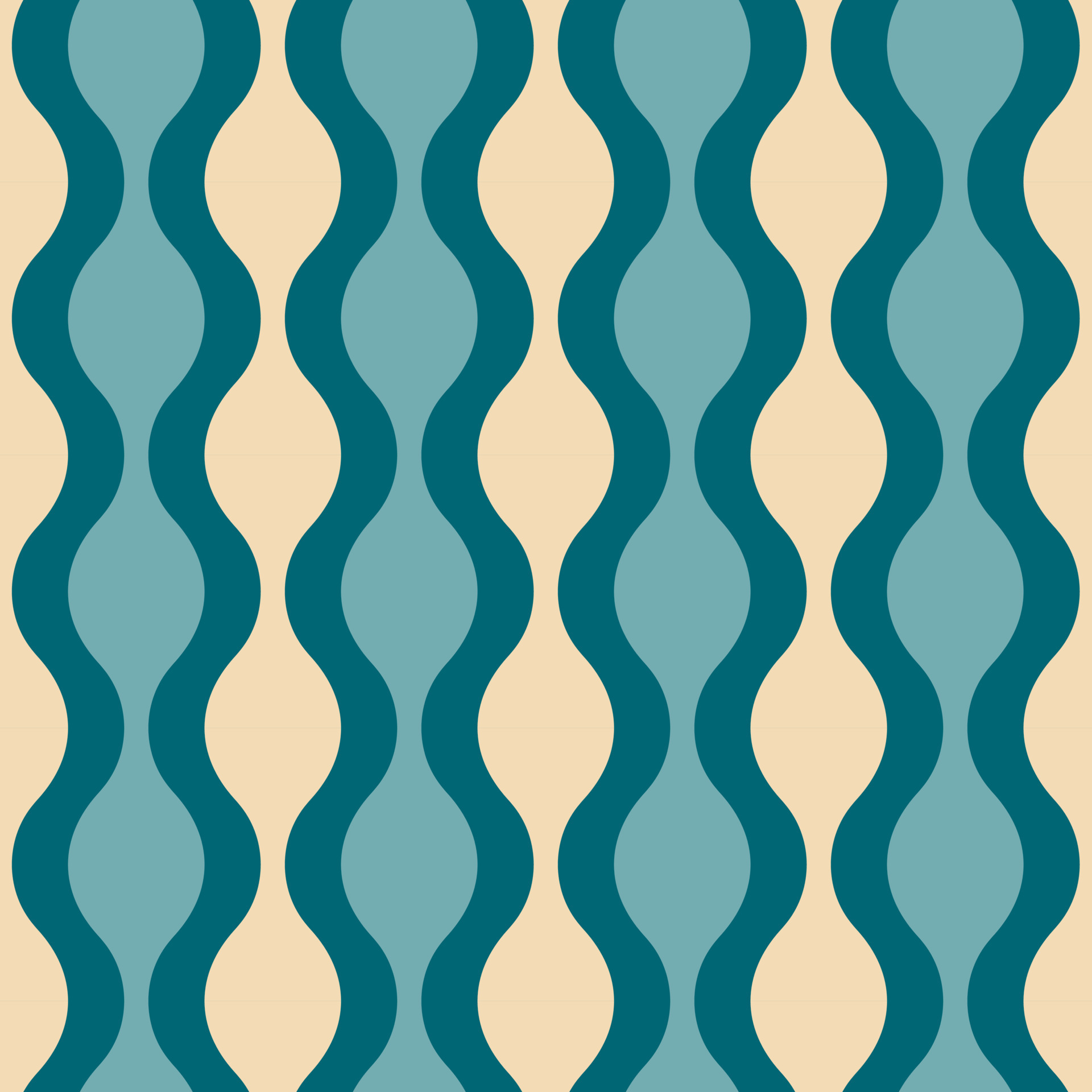The image depicts a repeating pattern spanning the entire canvas, set against a white or yellow background. This pattern consists of four vertical columns of identical designs featuring a wavy, S-curve motif. Each vertical strand resembles intertwined chains or beads, creating an optical illusion with alternating colors.

At the center of each segment is a light blue, circular shape that does not completely close, instead narrowing down before widening into another open circle. This core is bordered by a dark blue outline. The sections in between these curves create spaces filled alternately with light blue and cream colors, giving the design a sense of movement and depth. From top to bottom, each vertical column repeats this intricate pattern five times, making a visually engaging and detailed design that plays with color contrasts and symmetrical forms.